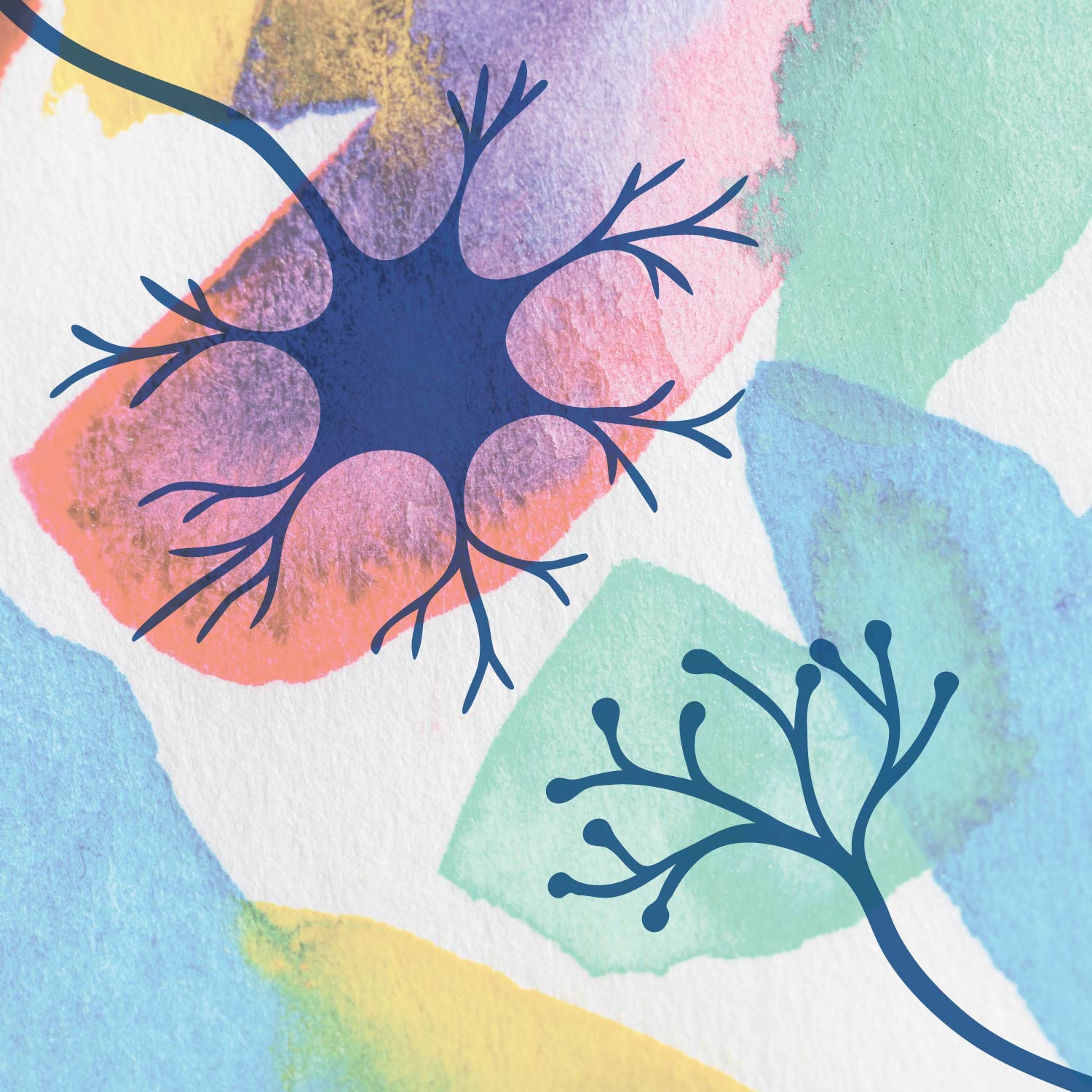This abstract painting features a complex interplay of tree-like and cellular structures against a vibrant watercolor background. Dominating the top left, a nucleus-like form with a star pattern takes center stage, rendered in solid purple and accompanied by a colorful backdrop of yellow, pink, and teal. At the bottom right, a plant-like figure with snaky, branch-like shapes reaches towards the center, surrounded by hues of green and blue. Both central figures are intricately detailed with small, beady terminal areas. The surrounding background is a blend of watercolor splotches in blue, pink, green, and yellow, creating a dynamic and multilayered aesthetic that contrasts with the solid, detailed foreground elements. White splotches intersperse the image, adding to its abstract and hand-painted charm.